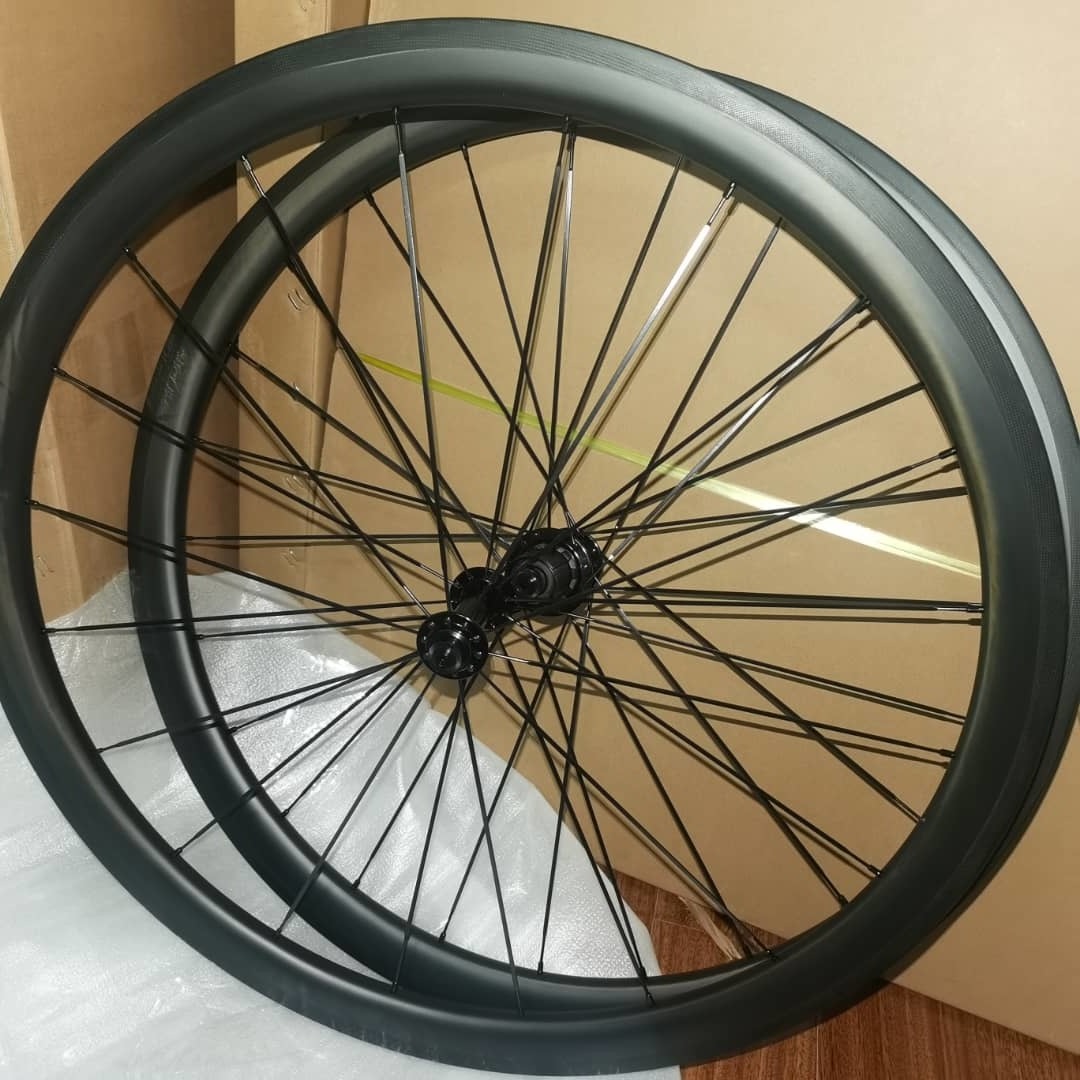This image features two solid black bicycle wheels, positioned with one slightly in front of the other, both leaning against a backdrop of three cardboard boxes. The wheels, with their black tires, spokes, and gears, stand on a hardwood floor of medium-toned brown. A light gray to white plastic bag or styrofoam sheeting is placed beneath the wheels, suggesting it as the packaging material for the tires. The cardboard boxes behind the wheels have notable details: one box with a visible strip of tape, another with visible staples, and a third box partially in view to the left. The scene is set in an indoor environment, likely a house, with various hues including tan, yellow, black, white, and brown present in the composition.